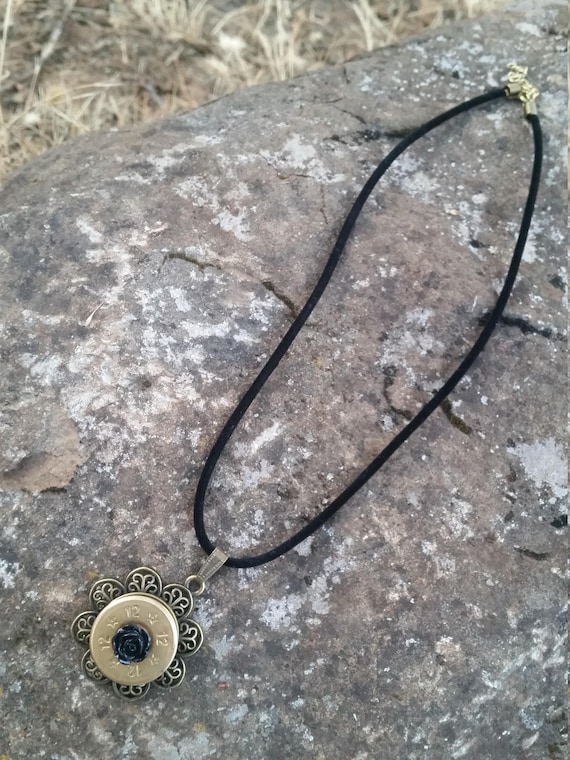This image showcases an intricate necklace, meticulously laid out on a weathered, grey stone slab. The stone's rough texture is complemented by the presence of some dying grass in the upper corners, hinting at an outdoor setting. The necklace features a black looped band with two gold clasps for fastening. The centerpiece of this accessory is a pendant designed to resemble a flower with multiple layers. The outermost layer consists of gold petal-like shapes, followed by a circular band with engraved numbers and stars. At the heart of the pendant lies a visually striking indigo rose, adding a touch of color to the predominantly metallic gold and black design. This beautifully crafted piece merges elements of old-world charm and delicate artistry, captured eloquently against the simplistic backdrop of the weathered stone.